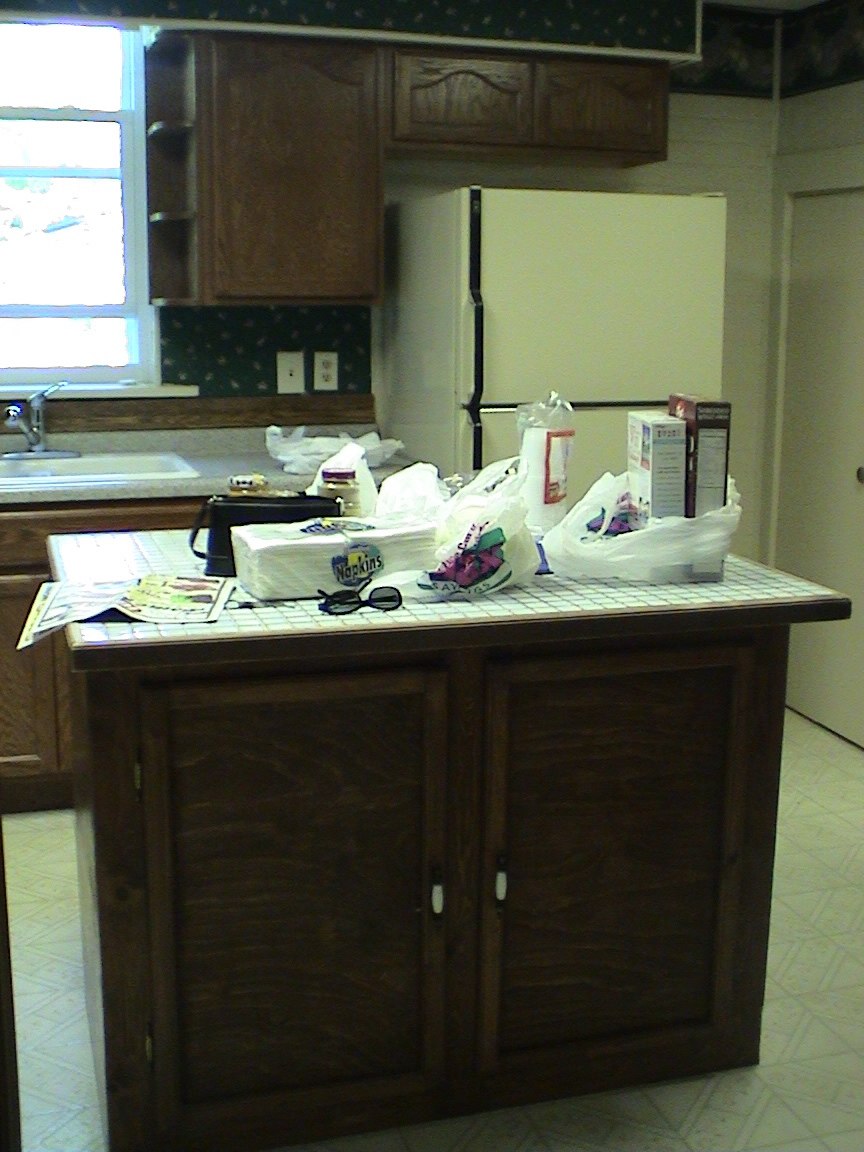This image showcases a bustling kitchen with a central focus on a small, dark brown kitchen island. The island, featuring two doors and a contrasting white countertop, is cluttered with various everyday items including a piece of newspaper, a purse, a bag of napkins, a pair of sunglasses, a bag containing two boxes, and another bag filled with what appears to be plastic lids. In the background, a beige two-door refrigerator stands tall, accompanied by an adjacent counter on the left-hand side. This counter bears additional clutter with several plastic bags strewn across it. Beside this counter is a kitchen sink located beneath a bright window that allows natural light to stream into the space. To the right of the window, a single-door, dark brown cabinet with slight shelving offers additional storage.